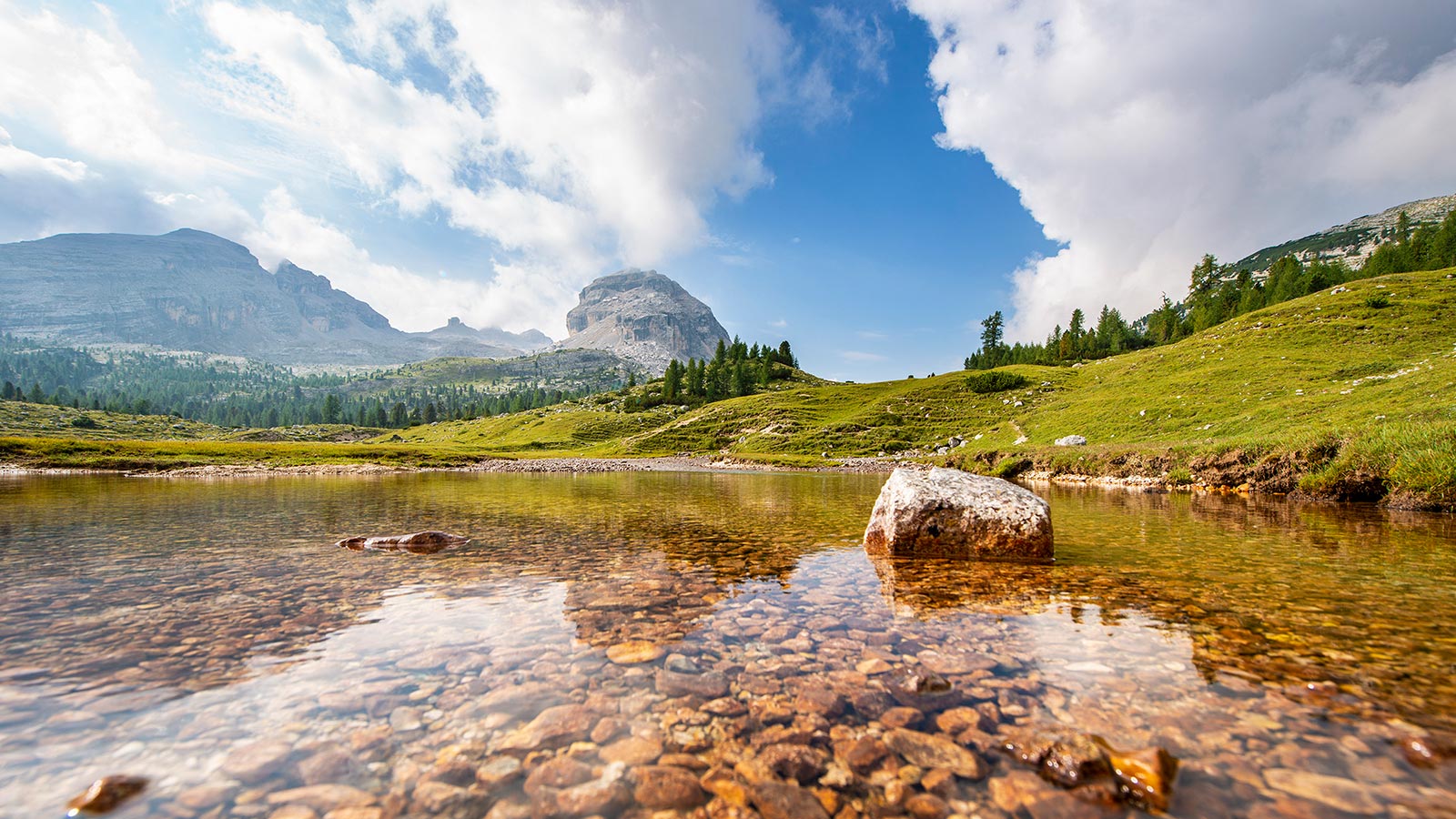This stunning photograph captures a serene natural landscape with remarkable clarity and detail. In the foreground, there is an expanse of crystal-clear, shallow water revealing an array of pebbles and various-sized brown rocks beneath the surface. The water is so transparent that every rock is distinctly visible, creating a mesmerizing view. One particularly large rock juts out from the water near the center-right of the image.

As your gaze shifts from the water, a rocky shoreline transitions into lush, green grassy hills. These hills are dotted with scattered evergreen trees, which appear more densely populated towards the left side of the image. Further into the background, a majestic gray mountain range rises, partially shrouded in mist and clouds, contributing to the ethereal atmosphere of the scene.

Above, a blue sky is visible, though partially covered by big, white clouds, especially prominent on the left and right edges of the photograph. The entire scene is bathed in a calm, tranquil light, evoking a sense of peace and natural beauty.